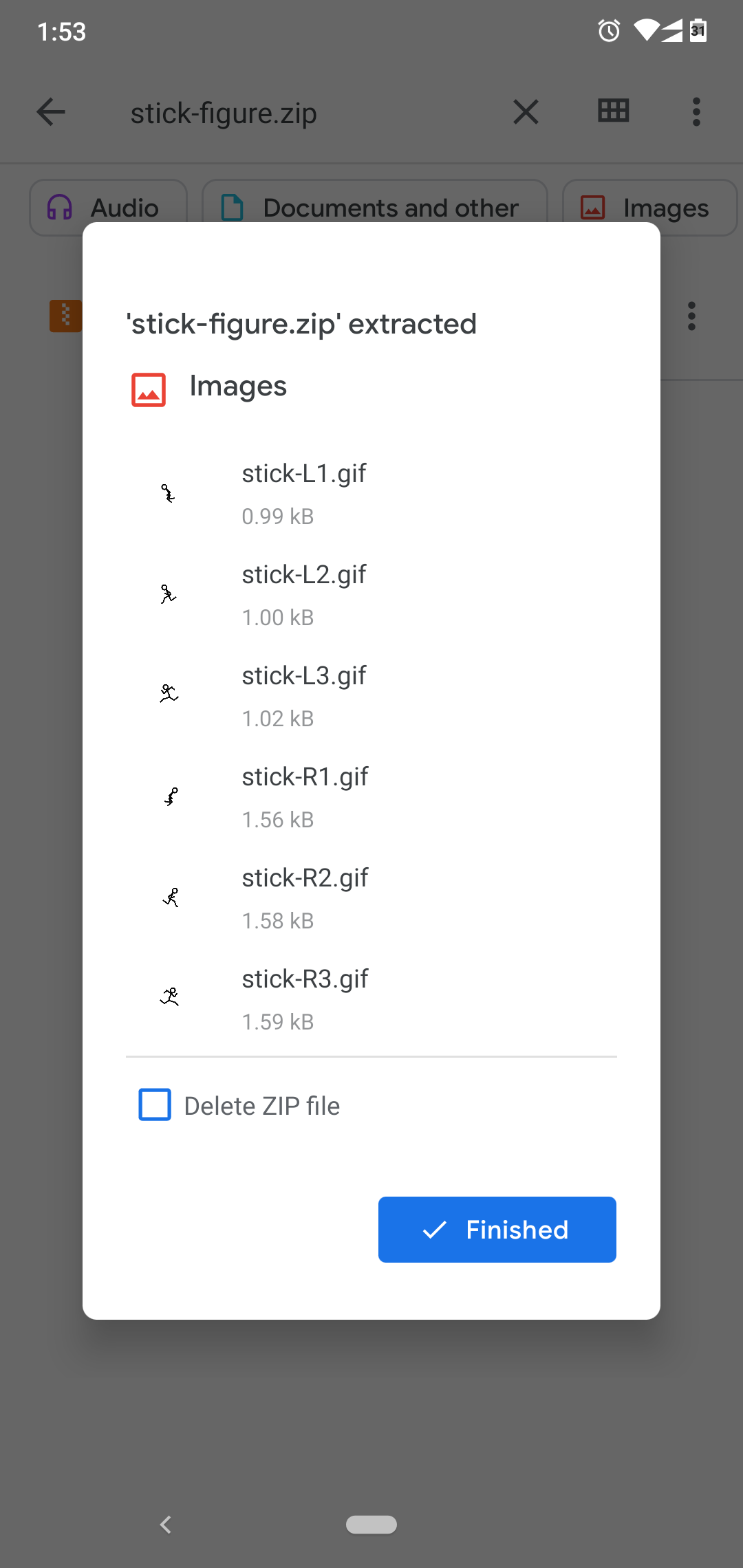### Detailed Caption

The screenshot depicts a zip file extraction interface on a gray background. The central area displays the contents of the "stick-figure.zip" file on a white background. At the top, the title "stick-figure.zip extracted" is prominently displayed. Below this title, there is a red-bordered box showing a thumbnail with two red mountains, indicating it contains image files.

The main section lists six files extracted from the zip archive. Each file is accompanied by an icon on the left side, featuring a black stick-figure either running to the right or the left. The files are named and sized as follows:
1. **stick.l1.gif** - 99.99 kilobytes
2. **stick.l2.gif** - 1 kilobyte
3. **stick.l3.gif** - 1.02 kilobytes
4. **stick.r1.gif** - 1.56 kilobytes
5. **stick.r2.gif** - 1.58 kilobytes
6. **stick.r3.gif** - 1.59 kilobytes

Below these files, a horizontal gray line separates the file list from an additional option. This option includes a blue checkbox next to the text "Delete zip file," allowing the user to remove the original zip file after extraction.

In the lower-right corner, there is a blue pill-shaped bar containing a white check mark and the text "Finished" in white font, indicating the completion of the extraction process.